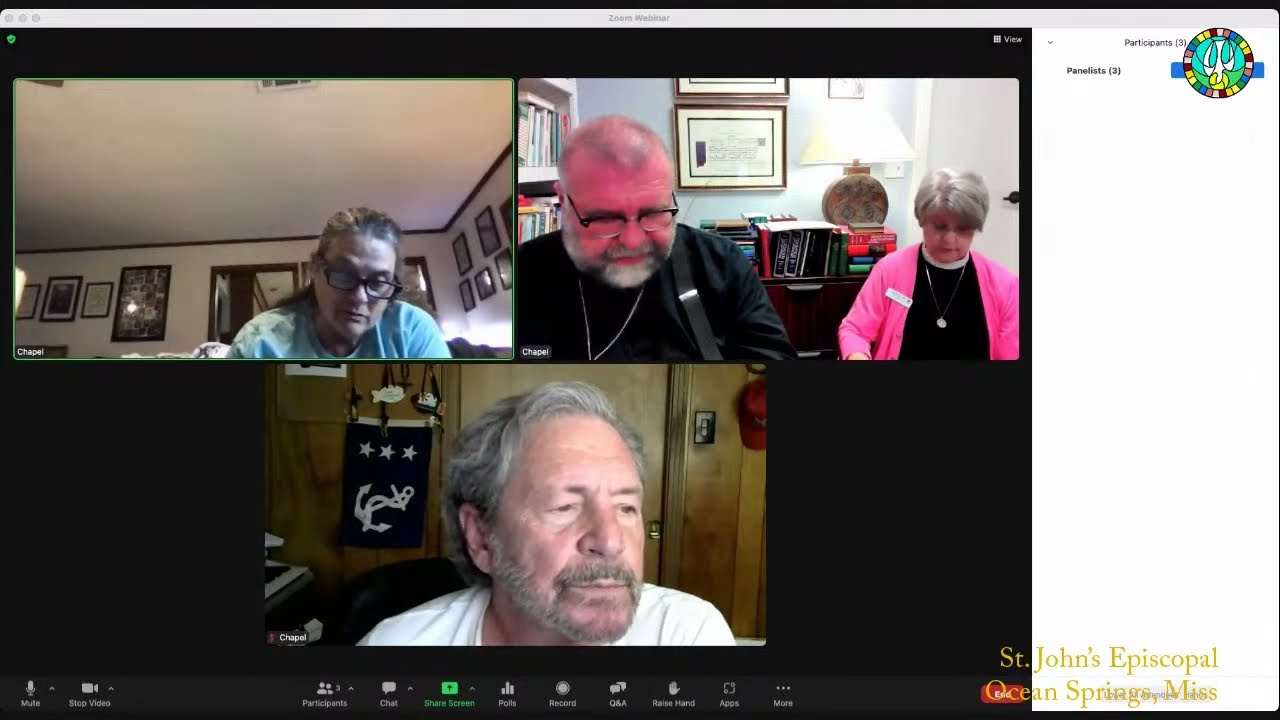This is a detailed screenshot of a Zoom video meeting featuring three participant windows, with St. John's Episcopal, Ocean Springs, Mississippi, labeled at the bottom right. The bottom window shows a man with gray hair and a gray beard wearing a white shirt, seated in an office-like room with wood paneling, a brown door, and a light switch. A red baseball cap hangs on the wall, and a flag with an anchor and stars is visible behind him.

The top left window features a woman with gray, long hair tied back, black-framed glasses, and a blue shirt. She's in a room with white walls and ceiling, adorned with many picture frames and an AC vent. A doorframe is visible behind her.

The top right window shows an older couple. The man, closer to the webcam, has short gray hair, a gray beard, and is wearing black glasses, a black shirt, and black suspenders. The woman next to him has short silver hair, black glasses, and is dressed in a black blouse with a pink cardigan, adorned with a white name tag. Behind them, there are bookshelves filled with books, picture frames possibly holding certificates, a table lamp, and a white door. 

At the bottom of the screen, typical Zoom controls are visible, including icons for mute, stop video, participants, chat, screen share, polls, record, Q&A, raise hand, and apps.